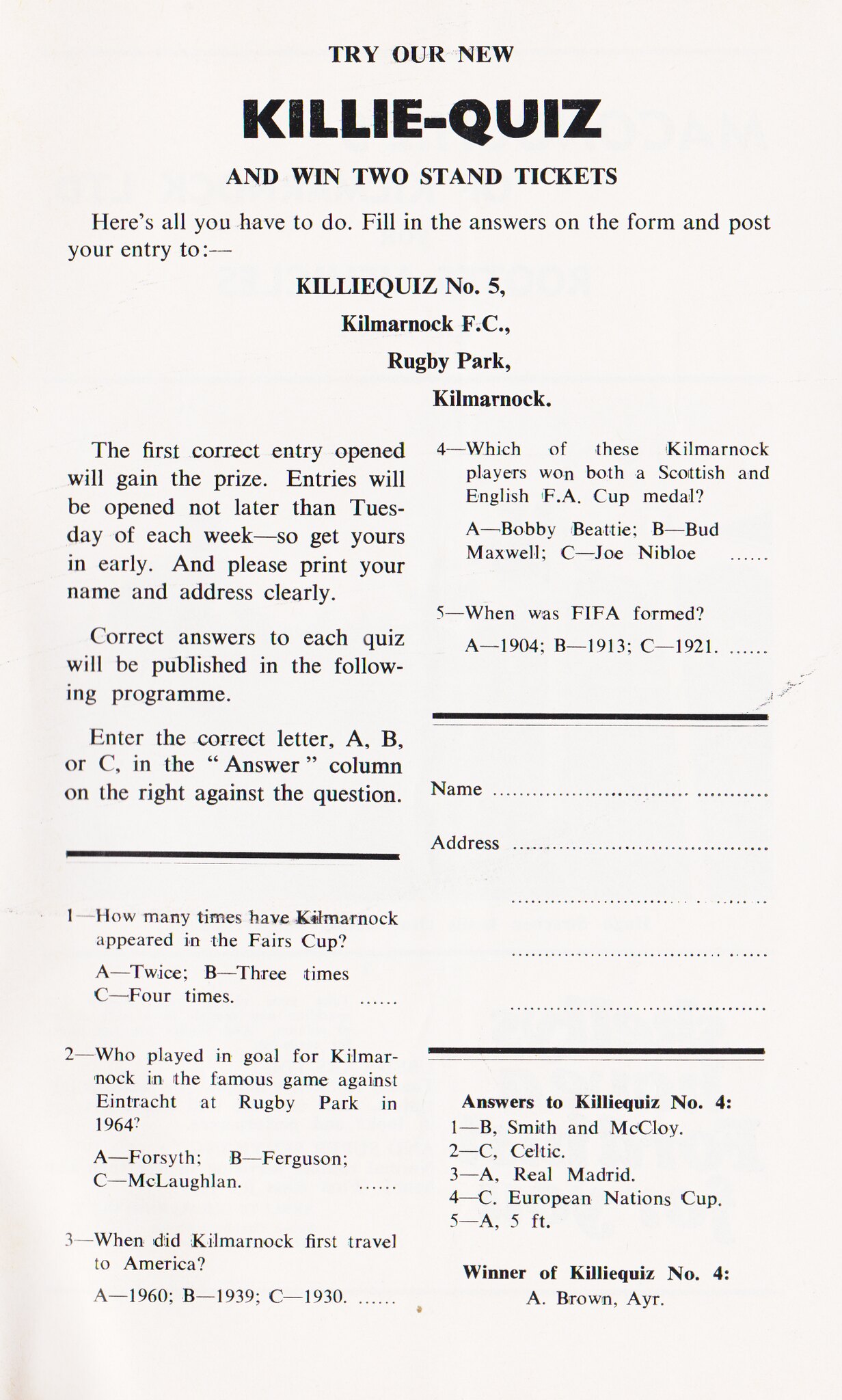This image is a page from a magazine or newspaper featuring a quiz to win a prize. At the top, it prominently says "Try Our New Kili Quiz" followed by "and Win Two Stand Tickets." The page, which has a white background with black text, instructs participants to fill in their answers on the form and post their entry to "Kili Quiz Number 5, Kilmarnock FC, Rugby Park, Kilmarnock." The content is divided into two main columns separated by thick black lines. 

On the left, there are several paragraphs explaining the quiz's directions followed by three quiz questions. The right column contains questions 4 and 5, followed by sections labeled for participants to write their name and address. Further down, below another thin black line, the quiz offers the answers to the previous "Kili Quiz Number 4," as well as the name of the previous winner. These details collectively guide participants through entering the quiz and provide a clear layout of the information needed for participation.